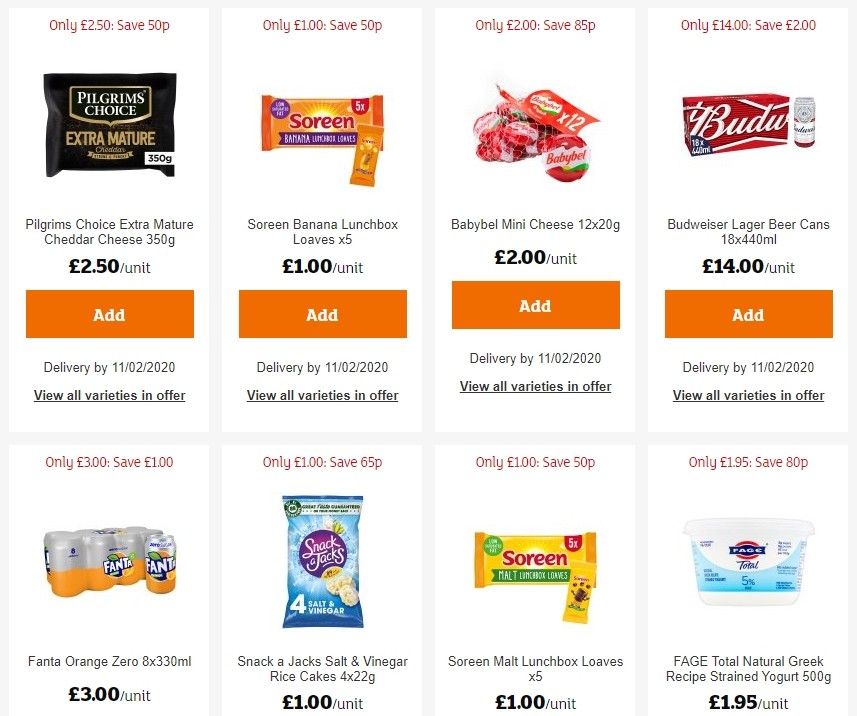The provided image appears to be from a UK-based online food ordering website, showcasing a selection of various food products with corresponding prices and options for adding them to a cart. 

The top row features the following items:
1. **Pilgrim's Choice Extra Mature Cheddar Cheese** - 350 grams, priced at £2.50 per unit. An orange button is available for adding this item to the cart. Additional details include delivery options and a link to view all varieties and offers.
2. **Serene Banana Lunchbox Loaves** - Pack of 5, priced at £1 per unit. Like the previous item, it includes an "add to cart" button, delivery options, and a link to view all varieties and offers.
3. **Mini Babybel Cheeses** - Pack of 12 (20 grams each), priced at £2 per unit. It also includes an add to cart button along with delivery options and a link to view all varieties and offers.
4. **Budweiser Lager Beer Cans** - Pack of 18 (440 milliliters each), priced at £14 per unit. This item features an "add to cart" button, delivery options, and a link to view all varieties and offers.

The bottom row contains the following items, although some images are partially cut off and lack add buttons:
1. **Fanta Orange Zero** - Pack of 8 (330 milliliters each), priced at £3 per unit.
2. **Snackajack Salt and Vinegar Rice Cakes** - Pack of 4 (22 grams each), priced at £1 per unit.
3. **Serene Malt Lunchbox Loaves** - Pack of 5, priced at £1 per unit.
4. **Fage Total Natural Greek Recipe Strained Yogurt** - 500 grams, priced at £1.95 per unit.

Overall, the website provides comprehensive options for selecting, viewing, and purchasing various food items, complete with pricing, weights, and additional details for a smooth online shopping experience.